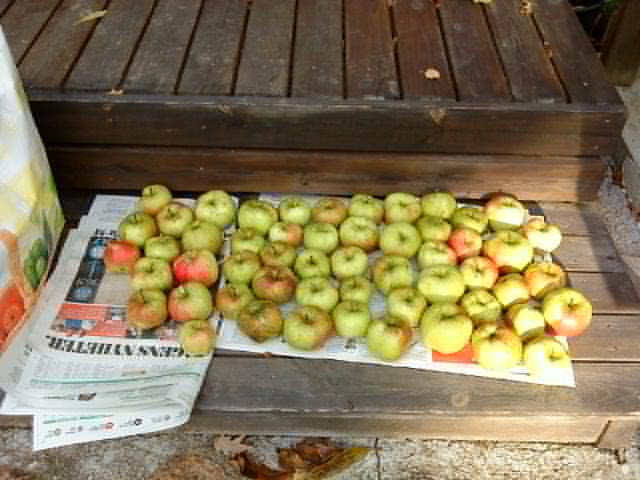An outdoor scene captures a rustic wooden deck with a lower wooden step beneath it, both surfaces showing signs of wear with some scattered dirt and fallen leaves. Below the deck is an asphalt walkway or parking lot. A large, colorful poster in white, red, orange, green, and yellow is affixed to the left side of the scene, partially behind a portion of a white feed or vegetable bag featuring a green pepper design. Laid out meticulously on about three layers of newspapers spread across the step are several dozen apples. The apples are primarily green, though some show patches of red, suggesting they are unripe. They are positioned with their stems facing up, some catching the sunlight while others remain in the shade, casting dappled light patterns. The sun illuminates the scene from the right front corner, highlighting both the apples and the weathered textures of the deck. The newspapers beneath the apples vary in their state, with some sections unfolded to provide a surface for the fruit. In the immediate foreground, brown and golden leaves augment the autumnal feel of the snapshot.